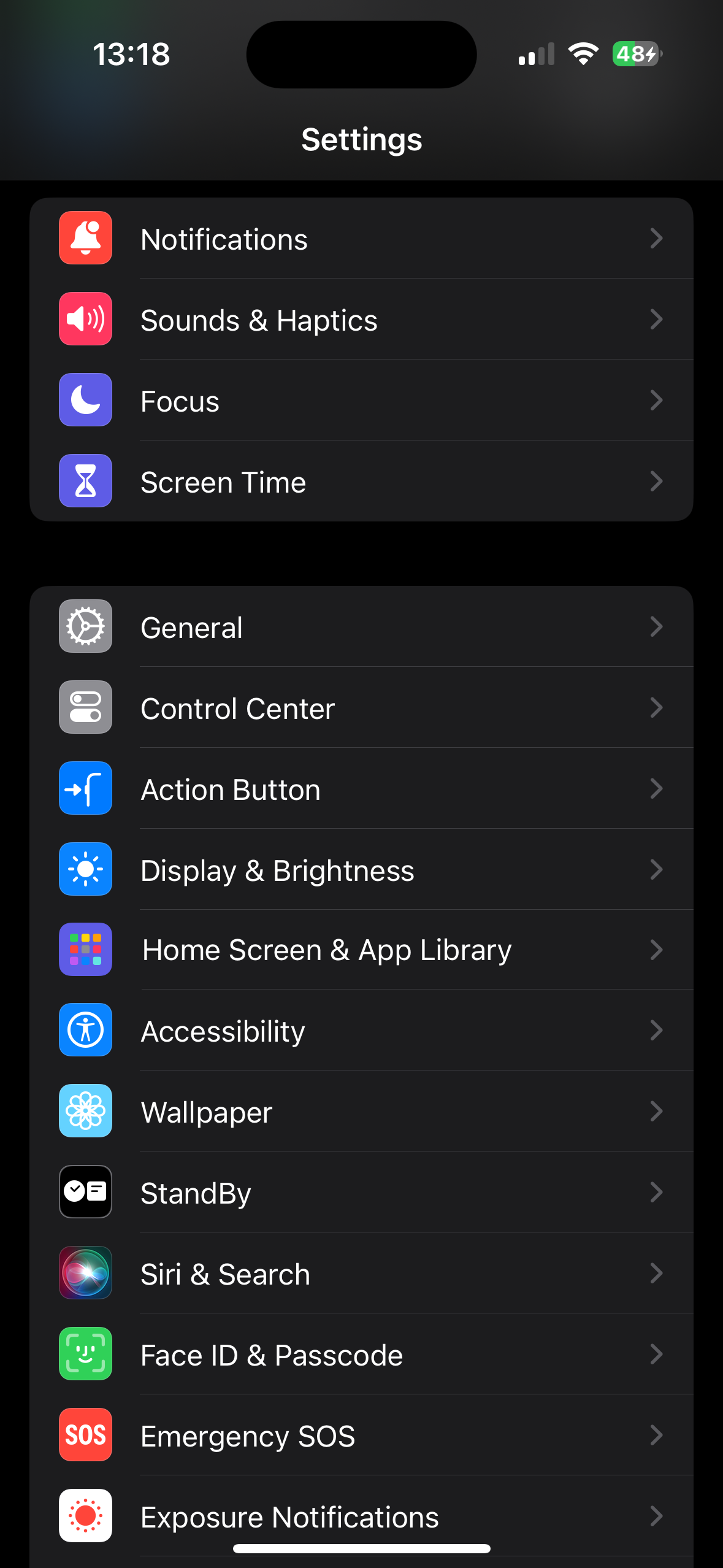The image captures a screenshot of an iPhone's settings menu displayed in dark mode. The background is black, with white text and various icons lining the left side, representing each setting. At the top of the screen, a pill-shaped cutout, characteristic of the newer iPhone models, is prominently visible. It separates some options and indicates an area for the front-facing camera and sensors.

The main settings options visible include "Notifications," "Sounds & Haptics," "Focus", "Screen Time," "General," "Control Center," "Action Button," and "Display." Each setting features a unique icon: "Focus" is represented by a crescent moon, "General" by a gear, and "Screen Time" by an hourglass. More options such as "Home Screen," "Accessibility," "Wallpaper," "Standby," "Siri," "Face ID," "Emergency SOS," and "Exposure" can also be seen. The "Siri" icon resembles a crystal ball, and the "Emergency SOS" icon is a red box with the letters "SOS" in white.

The clean, sleek interface and iconography are hallmarks of Apple's design philosophy, emphasizing functionality and ease of navigation.